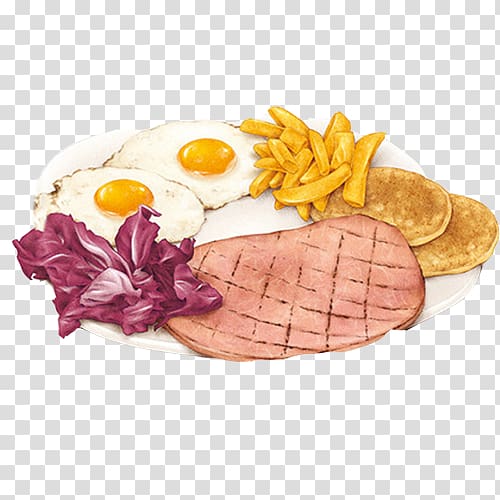This hand-drawn vector image of a breakfast plate, set against a white and gray checkerboard background symbolizing transparency, features a variety of foods meticulously illustrated with colored pencils. Central to the plate is a large slab of pink ham, grilled to perfection with visible lattice marks. Surrounding the ham are two golden brown, sunny-side up eggs with their yolks prominently displayed. To the right, a small handful of golden brown french fries adds a crispy contrast. Adjacent to the fries, two golden brown pancakes rest, completing the breakfast ensemble. Adding a touch of color, a handful of purple cabbage sits to the left of the ham. The white plate beneath these items enhances their vibrant colors, making this breakfast depiction detailed and appetizing.